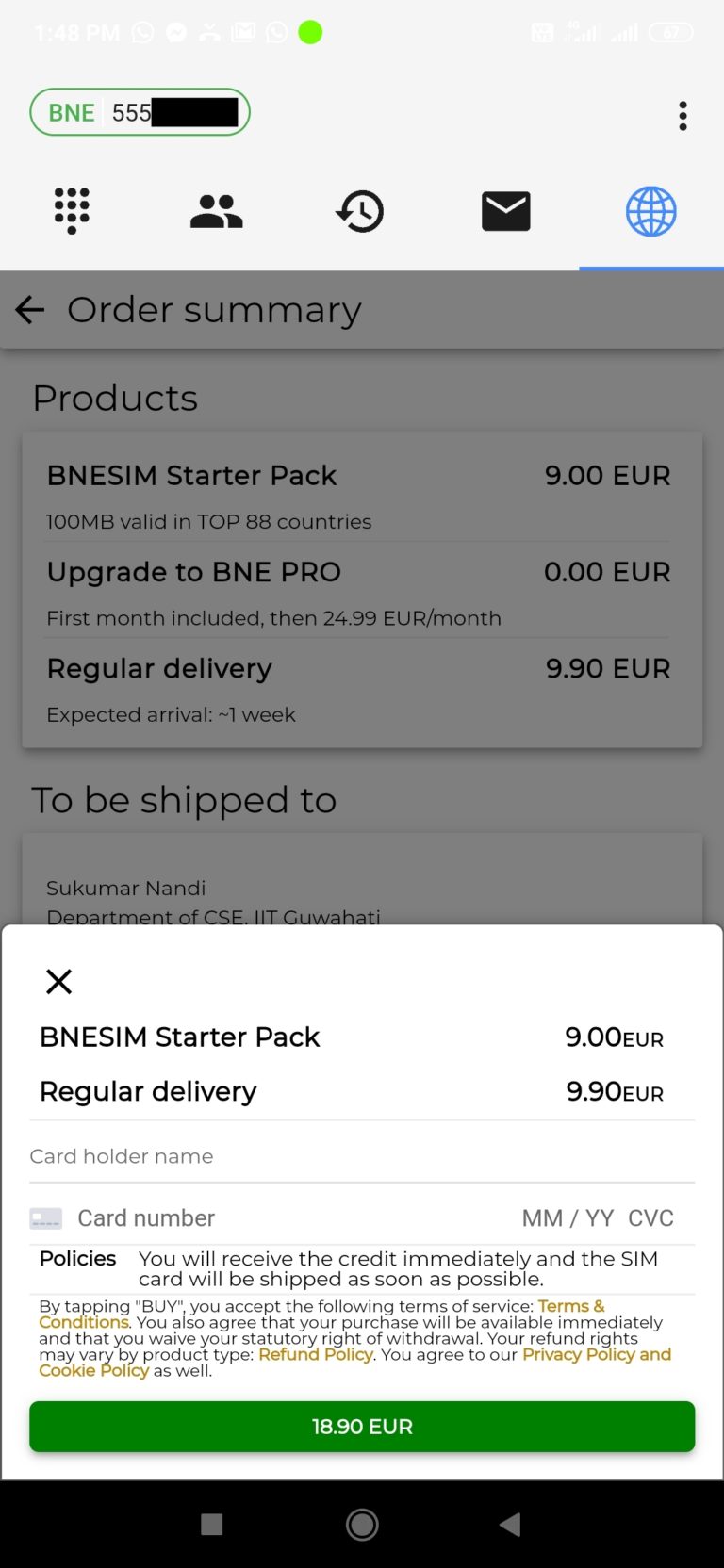**Detailed Order Summary:**

**Products Ordered:**
- **BNESM Starter Pack**: €9.00
  - **Features**: 100 Megabyte data, valid in top BB countries.

**Subscription Upgrade:**
- **Upgrade to Danny Pro**: 
  - **First Month**: Free of charge.
  - **Subsequent Months**: €24.99 per month.

**Delivery Details:**
- **Type**: Regular Delivery
  - **Expected Arrival**: 1 week
  - **Cost**: €9.90

**Shipping Address:**
- To: **Sukumar Nandi**
- Department of CSE, HT Guwahati

**Total Order Cost:**
- **BNESM Starter Pack**: €9.00
- **Regular Delivery**: €9.90
- **Total**: €18.90

**Payment Information:**
- **Card Holder Name:** [Blank]
- **Card Number:** [Blank]

**Policies:**
- **Credit Receipt**: Credit will be received immediately.
- **SIM Card Shipment**: The SIM card will be shipped as soon as possible.

**Additional Information:**
- **Terms and Conditions**: Followed by a Terms section.
- **Action Buttons**: A green button displaying "€18.90", along with Tab, Home, and Back buttons.